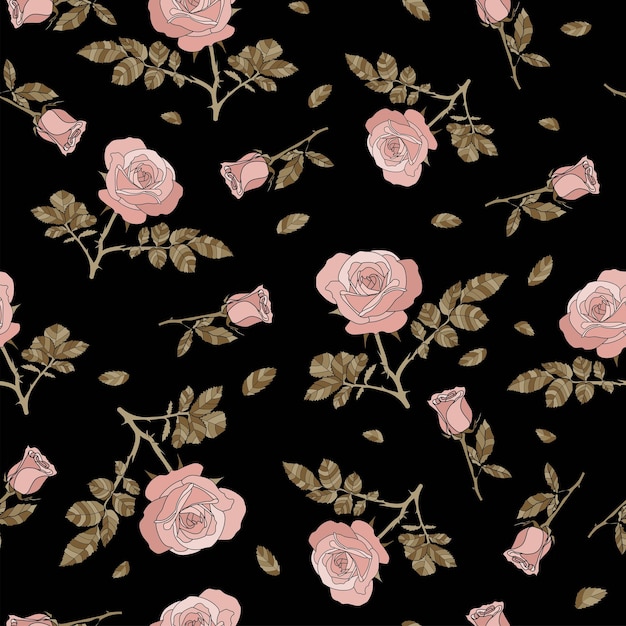This digital drawing features a striking composition of twenty pink roses of varying sizes and states of bloom, set against a solid black background. The petals of the roses exhibit an array of pink shades, ranging from very light to dark pink, and some include touches of white. Each rose is adorned with green, grayish-green, or light brown leaves, some of which are detached and scattered around. The roses are detailed with thorns, although not all stems display them. The arrangement of the flowers appears random, creating a dynamic yet harmonious visual impression. The overall scene suggests a sense of gentle falling or suspension, adding to the delicate beauty of the piece.